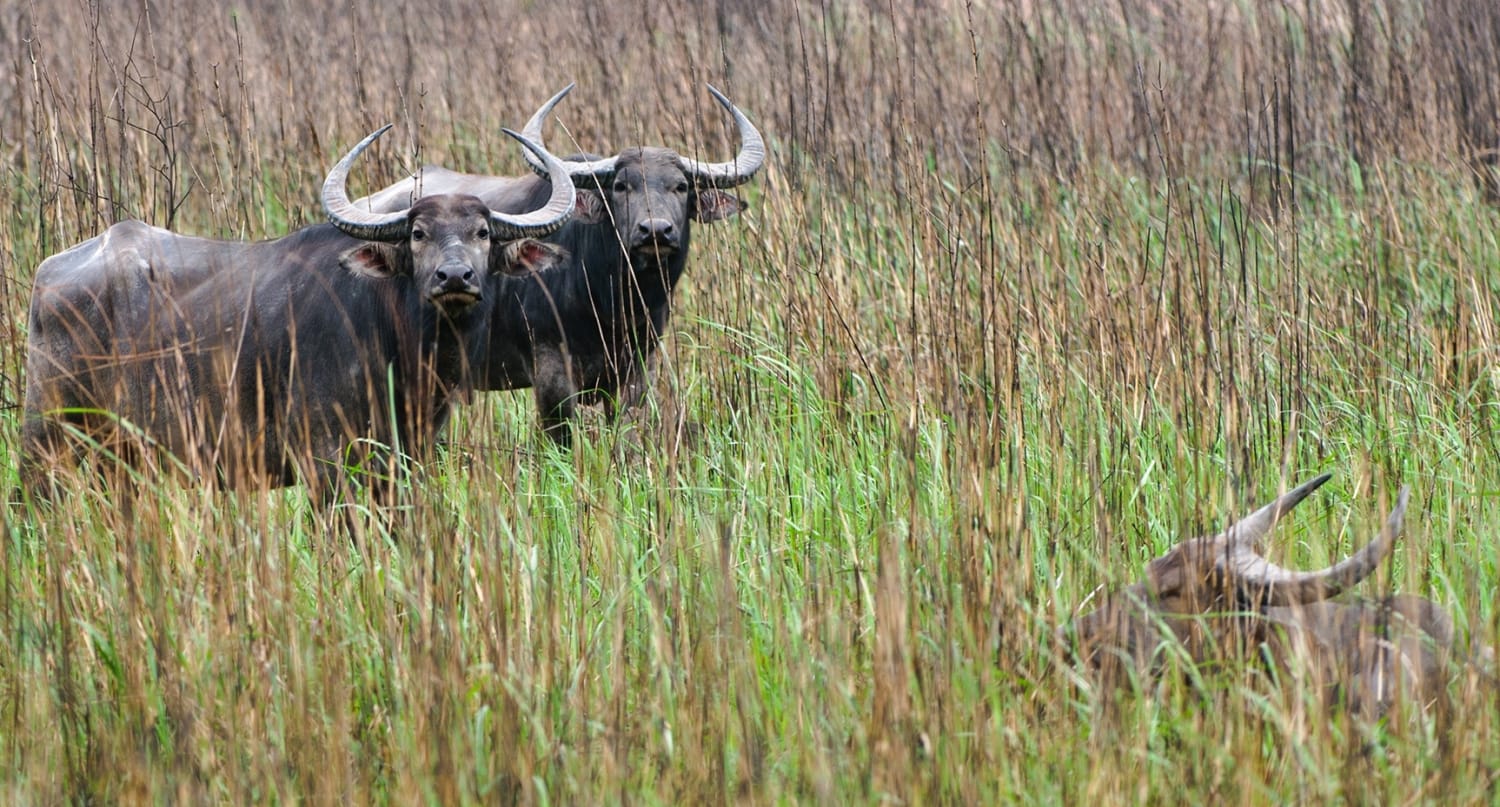A vibrant color photograph captures a panoramic view of a meadow adorned with tall, slender grasses in hues of green and brown. Amidst these swaying plants stand two imposing water buffalo, characterized by their muscular black bodies and large, gracefully curved gray horns that arch over their heads. Both buffalo are positioned side-by-side, staring directly into the camera with their outstretched ears framing their heads. Nestled in the grass in the foreground is a smaller, lighter brown buffalo calf, its shorter, less curved horns and profile view highlighting its youthful nature as it appears to be resting or sitting in the field. The scene exudes a serene wilderness essence with the harmonious blend of the animals and their natural habitat.